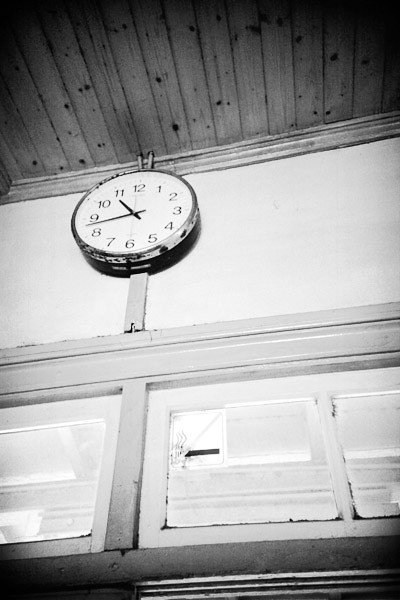This black and white photograph captures the interior of what appears to be an old classroom. Prominently displayed near the top of the wall, almost touching the light-colored wooden ceiling, is a vintage round clock. The clock features a black frame and classic design elements typical of older educational settings: black hands (both long and short), black numerals, and a white clock face.

The ceiling is composed of light-colored wooden planks that exhibit distinct grain patterns and bird's eye markings, adding a textured and organic feel to the room. The walls are painted white but are accented with wooden moldings, enhancing the room's period character. At the bottom of the image, three glass windows are visible, allowing light to filter into the otherwise stark and serene space. The overall atmosphere suggests a bygone era, evoking a sense of nostalgia and timelessness.